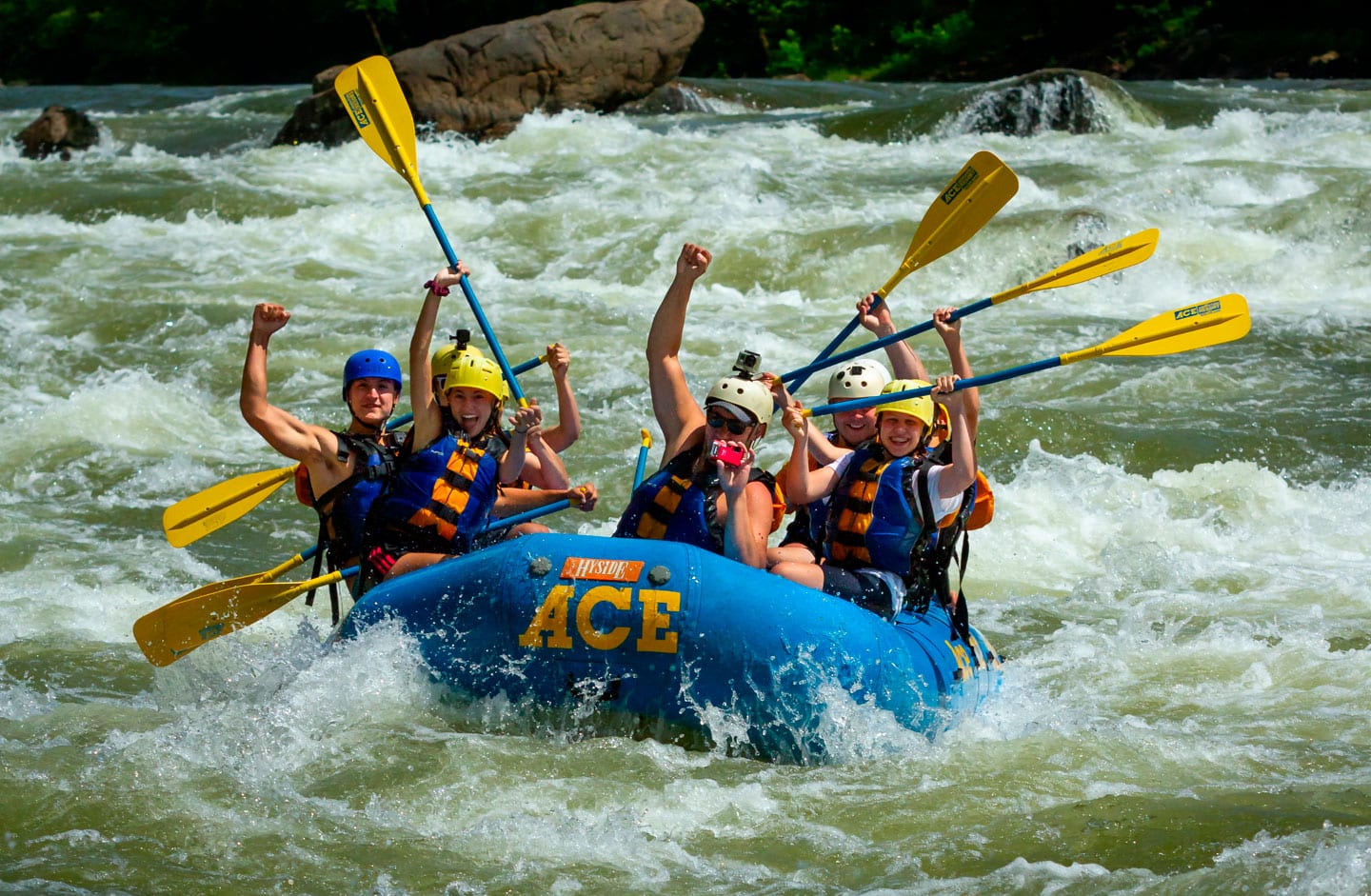In this vibrant daytime photograph, a group of young white-water rafters are captured amidst thrilling rapids. The action unfolds on a brackish green and brown river, with white-capped waves surging around their blue inflatable raft. The raft, prominently displaying the words "HI-SIDE" in white on a small rectangular sign, and the bold yellow letters "ACE" at its front, holds a diverse crew outfitted for adventure.

Each rafter dons a life vest distinguished by blue sides and orange centers, coupled with helmets in varying colors—yellow, white, and blue. Two helmets even sport mounted cameras; the central rafter's is a GoPro style, while the leftmost rafter's features a different type of attachment. Most hold aloft oars with blue handles and white blades, poised to navigate the churning water.

In the background, large stones jut out from the riverbank, amplifying the rugged scenery. A standout among these is a substantial stone on the left and a smaller one peeking through on the right. The rafters, seemingly exhilarated, strike a pose for the camera, with one at the front center wielding a red phone or camera. The image perfectly captures the essence of their high-energy river adventure under a sunny sky.